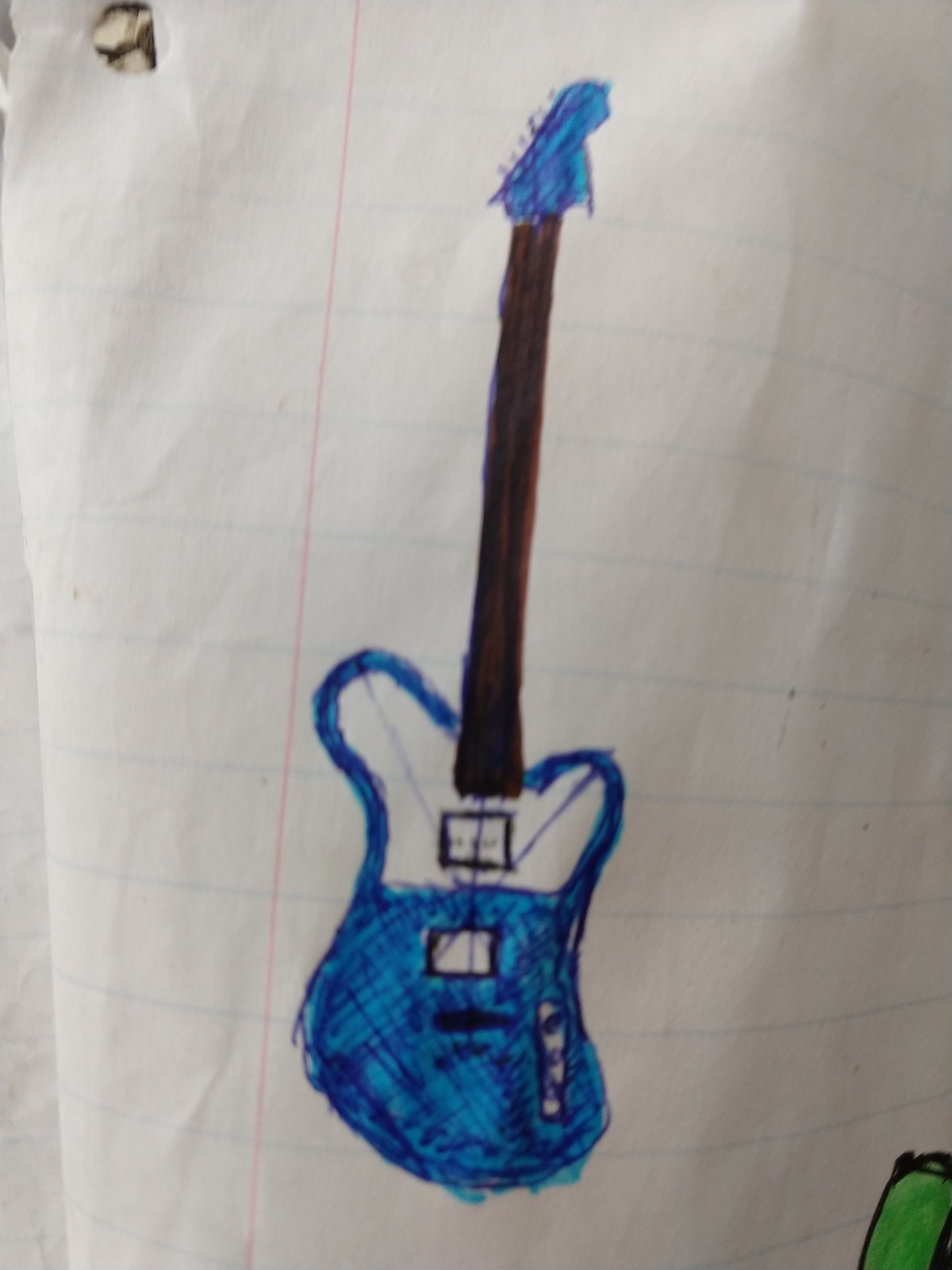This photograph captures a detailed drawing of an electric guitar sketched onto a piece of lined notebook paper. The notebook paper itself features the familiar blue horizontal lines and a single red vertical margin line, with the circular hole punch visible in the top left corner. The edges of the paper are slightly curled and folded over, adding a sense of texture to the image. The guitar drawing stands vertically in relation to the notebook paper, with the bottom of the guitar toward the lower part of the image and the head at the top. 

Notably, the guitar has a distinct blue body with white trim and two characteristic sound holes. The headstock and tuners, located at the top of the neck, are colored in bright blue. The neck of the guitar, extending from the body, is rendered in dark brown marker, appearing almost black due to the heavy layering. The drawing appears slightly out of focus, suggesting the camera was held too close when the photo was taken. Additionally, a sliver of another drawing, featuring a bright green rectangle with a black outline, can be seen in the bottom right corner of the image, but it is mostly cut off.